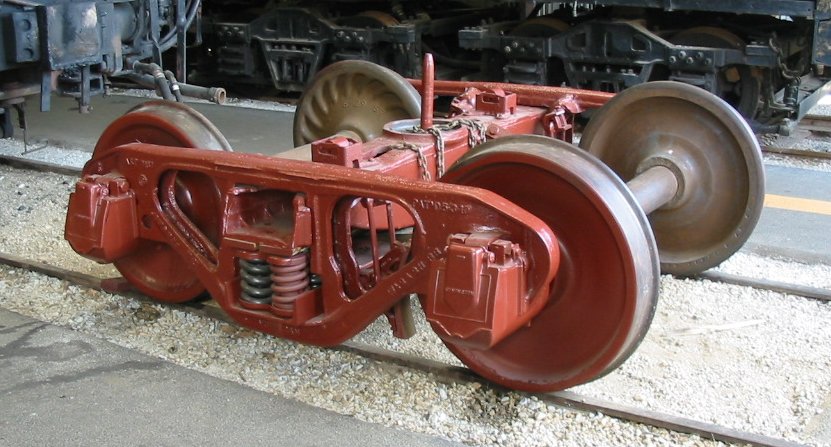The image captures a sunlit scene at a railway yard, displaying a close-up of four train wheels, unconnected to any carriages. These wheels feature silver-gray interiors with red exteriors, and are arranged in pairs on either side of the frame, linked by a cylindrical metal pipe. Between the wheels on each side, there's a distinctive red bar with a small circular mechanism at its center, which connects upwards to other train components. The wheels rest on parallel rails surrounded by white and gray gravel. In the background, partially visible, is a larger, black section of a locomotive, positioned on another set of tracks. Flanking the rails on either side are paved lanes, one featuring a yellow stripe. The scene is bathed in daylight, and a metal chain is faintly discernible towards the top of the image.